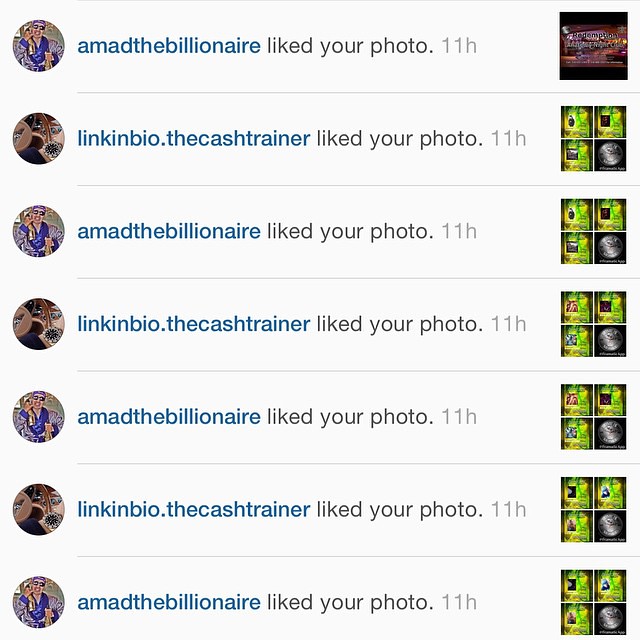The image is a screenshot of a social media notification window, likely from Instagram, showcasing a series of repetitive notifications. On the left side of the screen, there are small round profile pictures, acting as avatars, while on the right side, there are small snippets of photos that were liked. The notifications, stacked one below the other, detail that "Amanda the Billionaire" and "LinkedinBio.thecashtrainer" repeatedly liked the same photo 11 hours ago. The text reads: "Amanda the billionaire liked your photo 11 hours ago," and alternates with "LinkedinBio.thecashtrainer liked your photo 11 hours ago," spanning several lines. The repetition is notable and somewhat perplexing, indicating that the same two accounts have repeatedly liked the photo within the same 11-hour time frame. The visual representation on the right side of the screen shows the liked photo in a small, undistinguishable format, with some images containing mostly green and black colors. Overall, the notifications appear highly redundant and somewhat annoying.